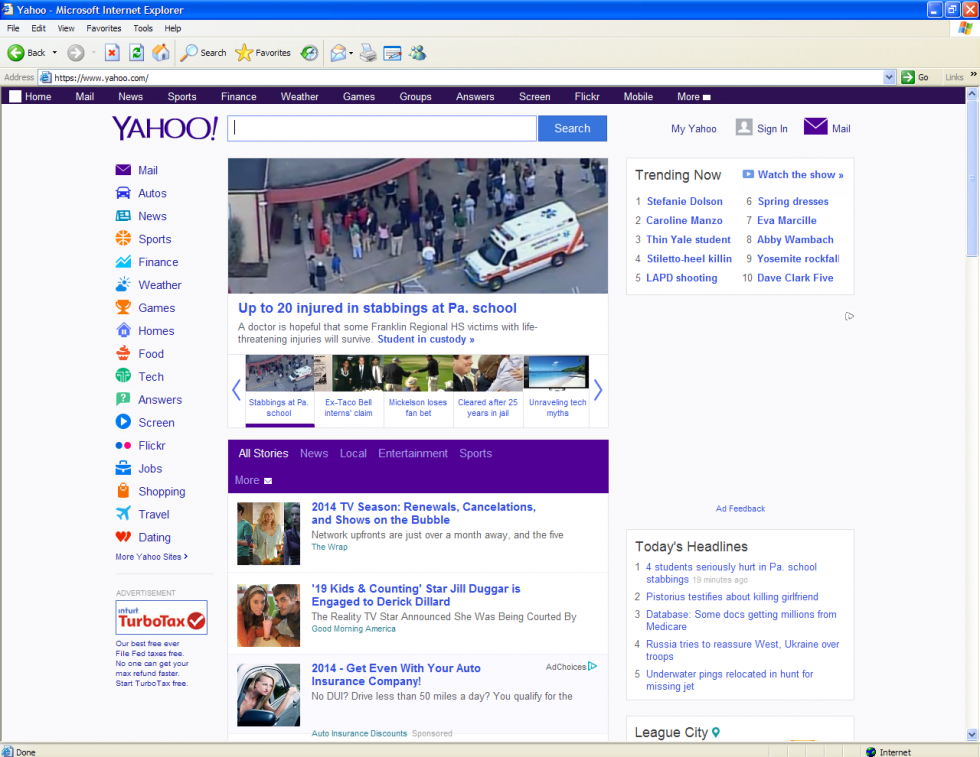Screenshot of a computer screen displaying the Yahoo homepage on Internet Explorer. The browser, Internet Explorer, features the standard interface with the minimize, maximize, and close buttons on the top right. The menu bar includes options like File, Edit, View, Favorites, Tools, and Help, as well as a back button and other navigation tools.

The Yahoo homepage is highlighted with its signature purple-themed navigation bar at the top, listing options such as Home, Mail, News, Sports, Finance, Weather, Games, Groups, Answers, Flickr, Mobile, and more. Below the navigation bar is the Yahoo search bar. 

Prominently displayed beneath the search bar is a news feature with an image of an ambulance in front of a store, captioned: "Up to 20 injured in stabbings at Pennsylvania School." Further down the page, a purple banner labeled "All Stories" precedes a list of headlines including updates on the 2014 TV season, such as renewals, cancellations, and shows on the bubble, and news about "19 Kids and Counting" star Jill Duggar's engagement to Derek Dillard. There is also an advertisement stating, "2014: Get even with your auto insurance company."

On the right side of the page, a "Trending Now" section lists popular topics, adding to the typical content one would expect from a Yahoo homepage.